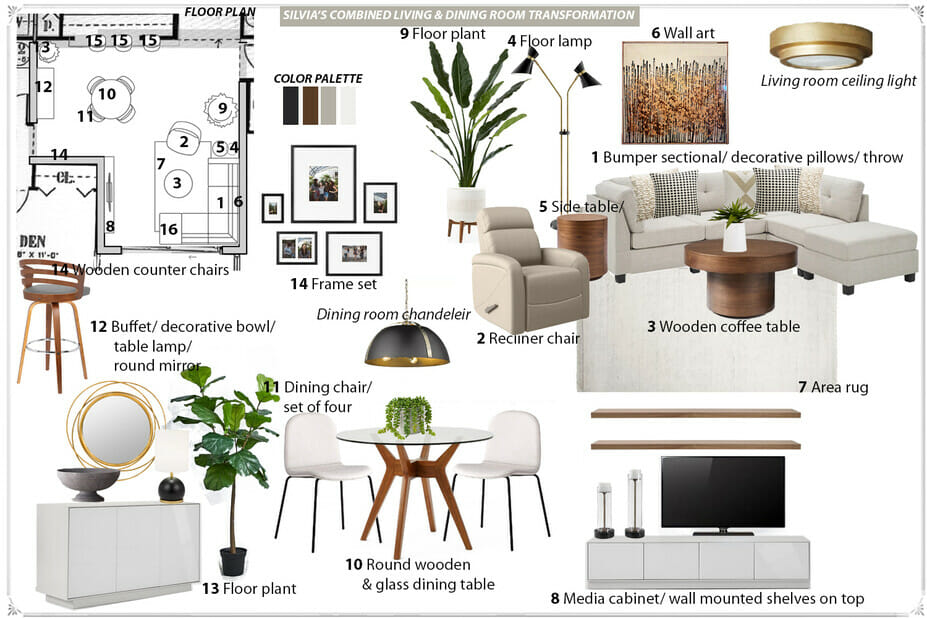A detailed floor plan of Sylvia's Combined Living and Dining Room Transformation is showcased prominently in the top-left corner of the image. It’s a blueprint layout of a single room, labeled with multiple numbers corresponding to various furniture items depicted alongside the plan. At the top, a small grey banner with white text announces the room's transformation. 

On the far left, there's a picture of a wooden counter chair labeled "14 Wooden Counter Chairs," alongside images of a buffet, decorative bowls, a table lamp, a round mirror, and a side table marked with specific numbers that match those on the floor plan. Additional items include a floor lamp, wall art, a living room ceiling light, a bumper section, sash decor, throw pillows, a wooden coffee table, an area rug, and a round wooden and glass dining table. A variety of colors like greens, yellows, reds, browns, tans, whites, beige, black, and gray are used throughout the design.

The furniture items are spread across the white background, including beige chairs, a beige couch, a beige rug, a brown wooden table, white chairs, a white buffet, and a white media cabinet. Some items such as the buffet, floor plant, and dining room chandelier are not in numerical order but are arranged according to their location on the floor plan, which is numbered up to 16.